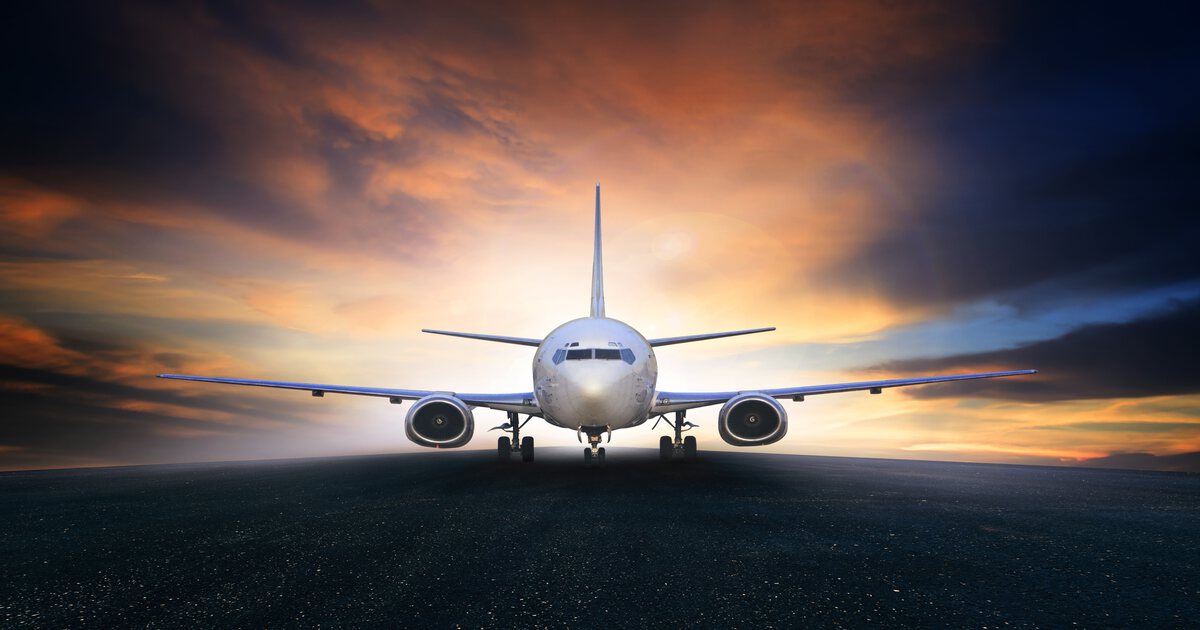The image captures a striking scene of a large commercial jetliner, with two engines mounted under its wings, facing directly towards the viewer. The aircraft, a passenger airplane in white and light blue, is either poised on the runway or appears as though it is coming at you at great speed, ready to take off. The plane is framed by its extended landing gear, under which the ground appears dark and black. The background showcases a dramatic interplay of colors: the sky behind the plane transitions from a bright, white glow in the center, suggesting the brilliance of a rising or setting sun, to hues of yellow, orange, red, and purples. Along the horizon and in the outskirts, the sky deepens into dark blue and eventually black, dotted with the faint pinpricks of city lights below, indicating it might be early morning or late evening. The sun, perched directly behind the plane, illuminates the scene with varying shades of light breaking through the clouds, creating an impression of motion and speed. This juxtaposition of the imposing jetliner and the vibrant, gradient sky creates a visually captivating image.